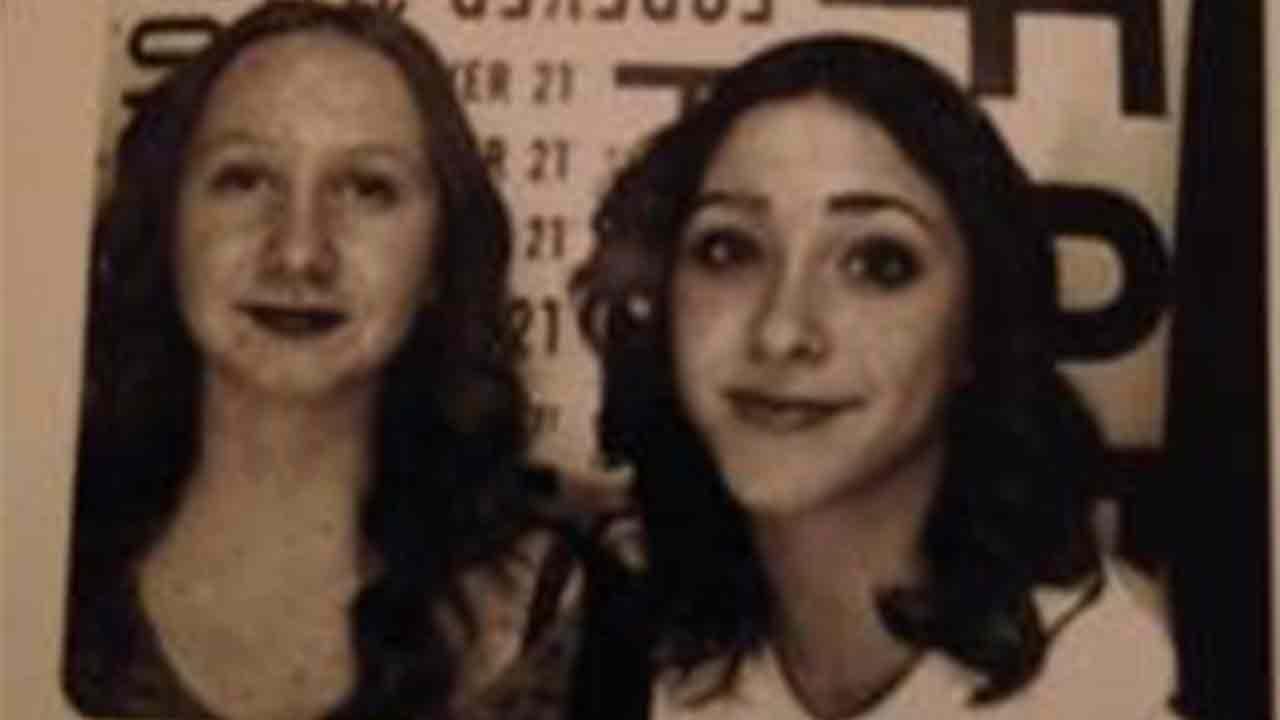This black-and-white photograph appears to be a vintage family photo, likely taken in the 1960s or 1970s, though it could also be from an earlier period such as the 1920s. It features headshots of two young women, possibly sisters or friends, standing close together. Both women have dark hair, are semi-smiling, and appear to be in their mid-to-late twenties or early thirties. Behind them is a partially obscured sign with the number "21" repeated multiple times, though the rest of the text is indecipherable. The photo is somewhat blurry and the edges are cut off, adding to its antique charm and mystery.